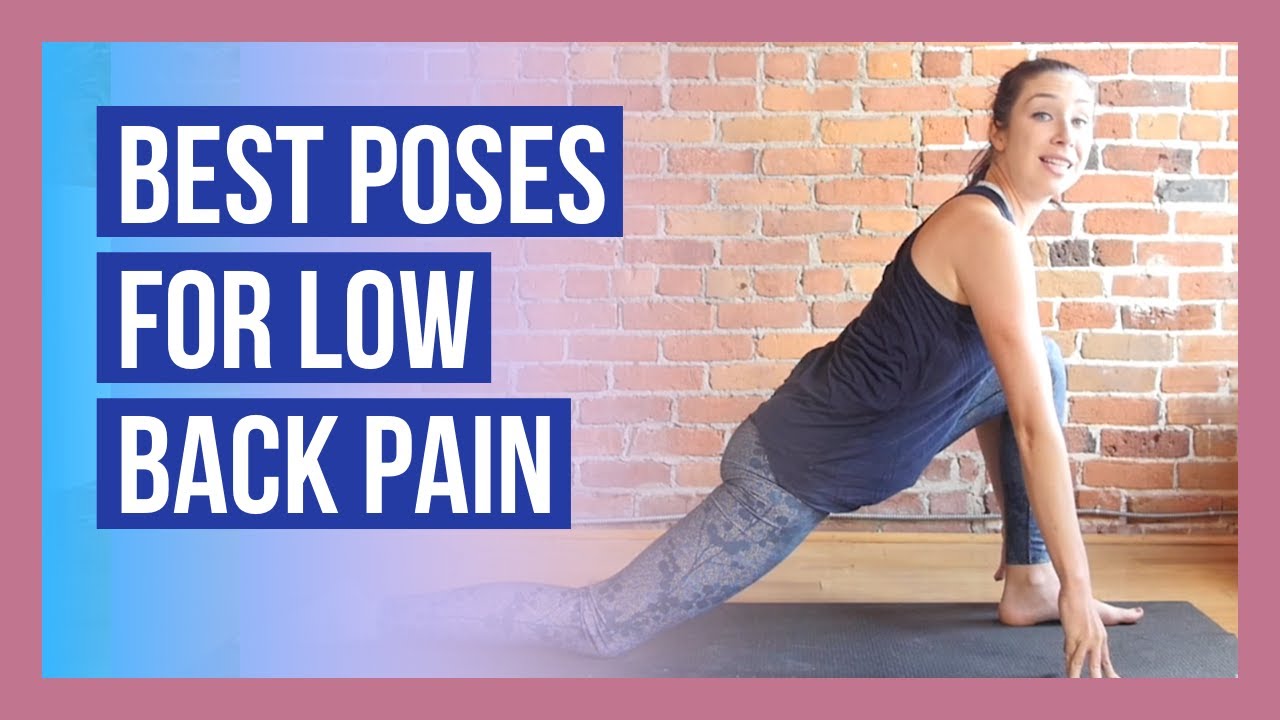The image depicts a young Caucasian woman, likely in her 20s, performing a yoga pose designed to alleviate low back pain. She is kneeling on a black yoga mat with one leg bent forward and the other fully extended behind her. Her light blue leggings feature a deeper blue floral design, and she is wearing a sleeveless, navy blue workout top. The woman, who has long brown hair tied back into a ponytail, is looking straight at the camera with a slight smile. The backdrop of the scene includes a red brick wall and a wooden floor. To the left of the woman, there are three bright blue boxes with white text that read “Best poses for low back pain,” while the entire image is encased in a light pink border.